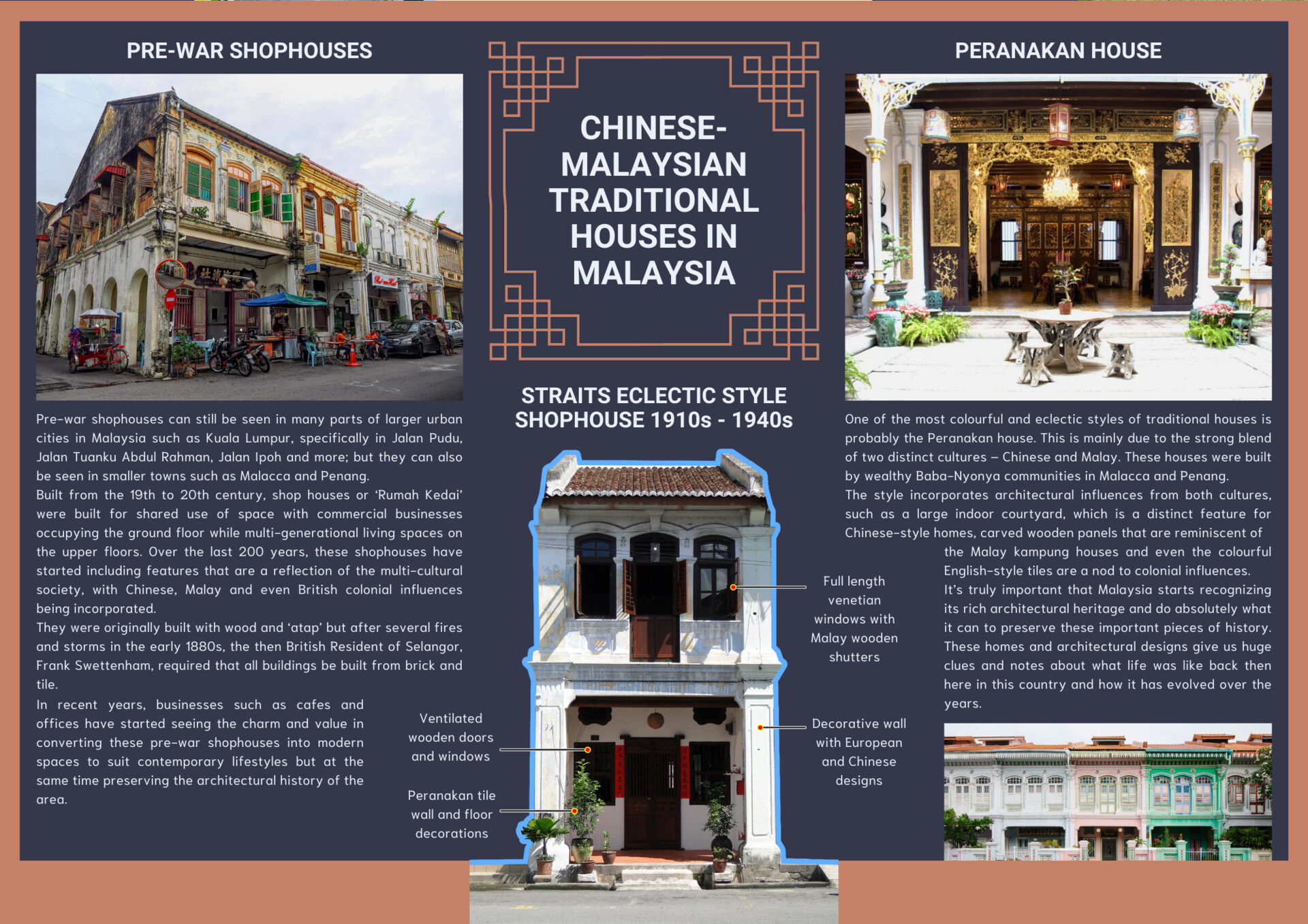The image is a richly detailed infographic showcasing various traditional Chinese-Malaysian houses in Malaysia, with an emphasis on pre-war shop houses and Peranakan houses. The infographic is divided into multiple sections featuring images and descriptions of these architectural styles. 

In the upper left corner, there's a depiction of pre-war shop houses, characterized by their multi-story structure lined up along a street reminiscent of a typical urban setting. These buildings feature intricate red and orange decorative trims around the white facades, and the presence of vehicles like carriages, cars, and motorcycles, along with caution cones, evoke a bustling city atmosphere.

On the opposite upper right corner, a detailed image of a Peranakan house is presented. This house is noted for its ornate design, including a squared archway richly adorned with gold, black, and white decorative elements. The Peranakan house is described as having an open space type of home layout.

Centrally positioned towards the bottom, the image showcases a two-story Straits eclectic style shop house from the 1910s to the 1940s. This building style is marked by full-length Venetian windows with Malay wood shutters, walls decorated with a blend of European and Chinese designs, and ventilated wooden doors and windows. The colors mentioned in the infographic include pink, green, white, red, brown, blue, and salmon, adding to the vibrant depiction of these traditional houses.

Accompanying the images are paragraphs of text that offer descriptions and historical context, emphasizing the eclectic architectural styles and cultural significance of these traditional Malaysian homes. The entire layout is encased in a brown border, resembling a meticulously designed brochure.